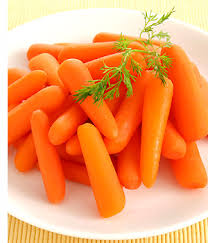The image is a zoomed-in photograph, likely a thumbnail or ad insert, featuring a plate of vibrant baby carrots. The carrots, exhibiting a range of shades from light yellow to darker orange, are arranged in a disordered heap on a bright white circular plate. A delicate sprig of green herb, possibly dill or parsley, is placed on top of the pile, adding a touch of freshness. This plate sits on a textured, ribbed yellow background that is more defined in the foreground and becomes blurry towards the back, giving a slight depth to the image. Though the exact purpose of the image is not specified, it could be an advertisement or a menu insert for a restaurant, highlighting the simplicity and attractiveness of the dish.